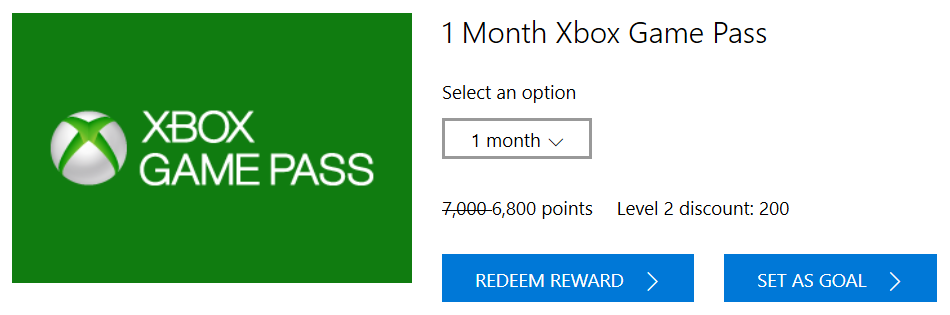The image appears to be a screenshot, possibly taken from an Xbox website, showcasing a promotional offer for the Xbox Game Pass. The layout begins on the left-hand side with a green rectangular section featuring the Xbox Game Pass logo. The logo itself includes the Xbox emblem, which has a green "X" on the inside and a silver outline.

At the top center of the image, the text reads "One Month Xbox Game Pass." Directly below this, there's a prompt that says "Select an option," followed by a rectangular box with gray borders. Inside this box, the text "One Month" is displayed alongside a drop-down arrow.

Below the selection box, the original price of "7,000 points" is shown, but it is struck through, indicating a discount. The updated price of "6,800 points" is then listed. To the right of this pricing information, there's a note that says "Level 2 Discount: 200."

Further down, there are two elongated rectangular buttons. The first button, colored blue, contains the text "Redeem Reward" with a right-facing arrow next to it. The second button, also blue, is labeled "Set as Gold" and similarly features a right-facing arrow. The background of the entire image is predominantly white, providing a clean and uncluttered appearance.

Overall, the image is a focused segment from the Xbox website, detailing a one-month subscription offer for the Xbox Game Pass, complete with discounted pricing and options for redemption or additional features.